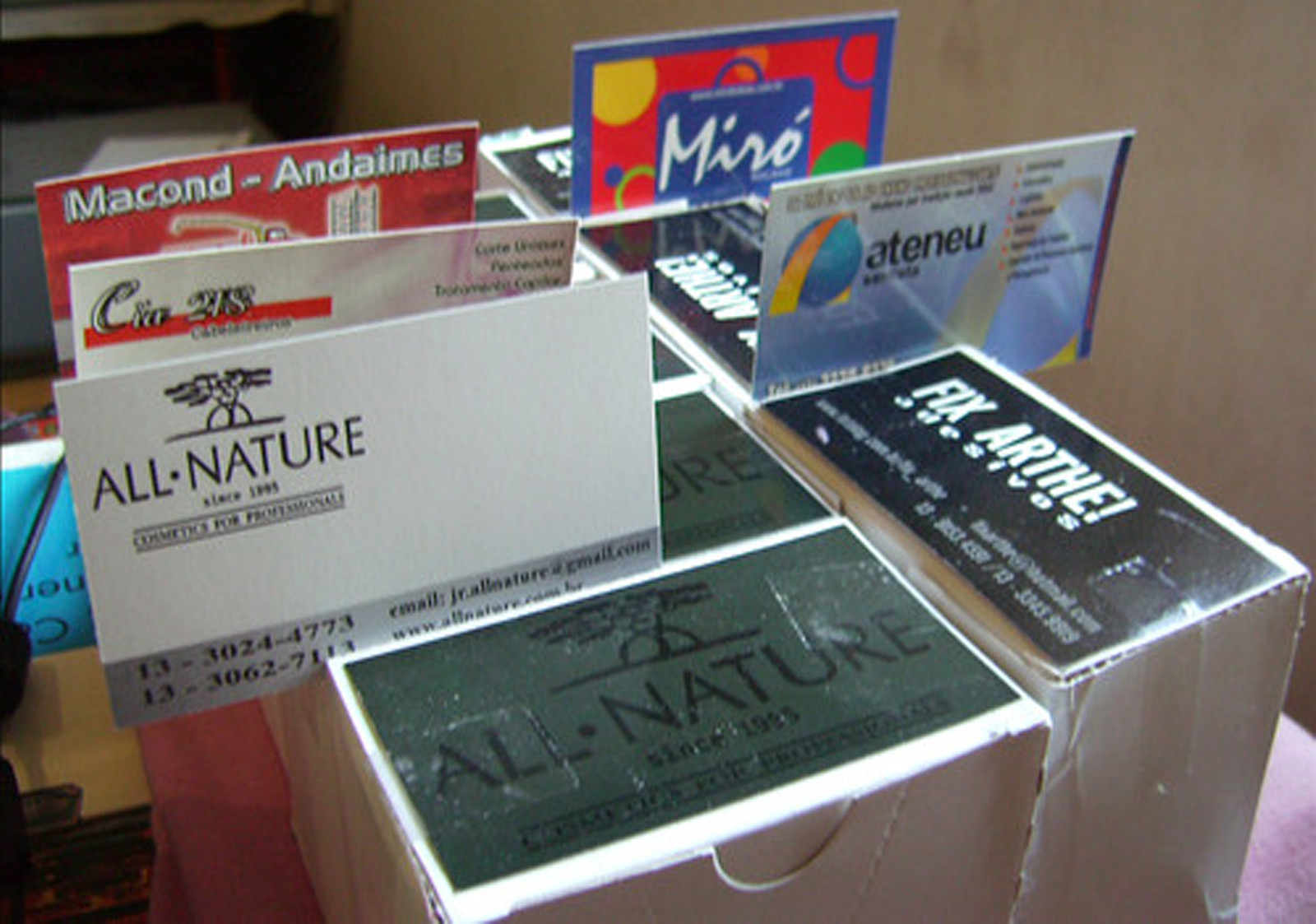This full-color, horizontal photograph showcases an array of brightly colored boxes organized in a row. Each box features a variety of business cards taped to their exteriors, all featuring different logos, colors, and languages. The detailed business cards include labels such as "All Nature Since 1935," "Macond Adonimus," "Fixarth!" with two other signs labeled "Attenue" and "Miroir" atop the stacked boxes. The "All Nature Since 1935" label is repeated multiple times, including on a white perpendicular sign that also lists an email address and phone numbers. The photograph includes boxes and cards with names like "SIA 218," "Macond," and several in foreign languages, with at least eight or nine distinctly different business cards visible, each with unique logos and color schemes. Some logos are vibrant blue or feature blue globes with yellow accents. It’s unclear from the image what products these boxes contain; there are no specific indications.